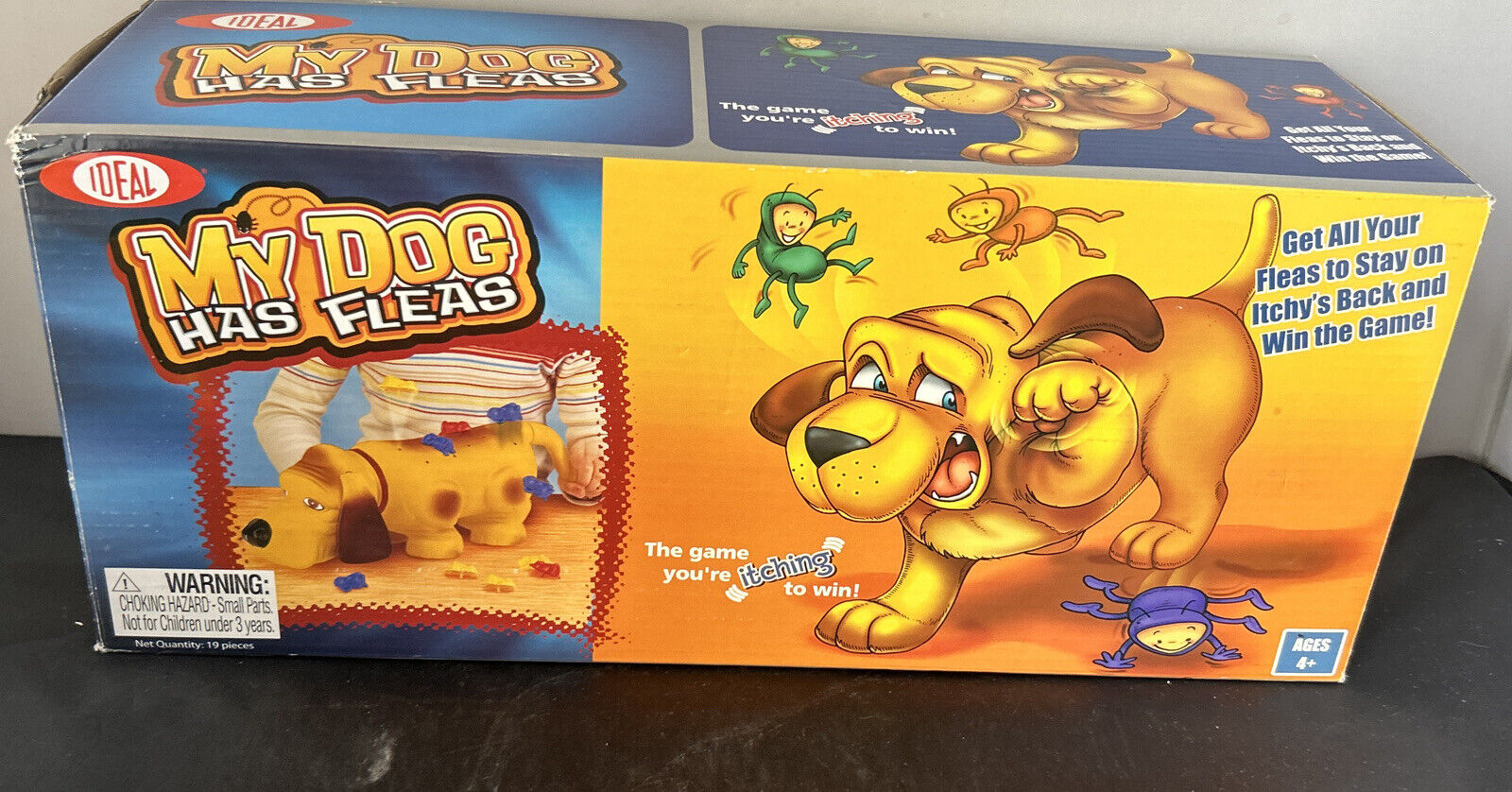The image shows a long rectangular box for a toy game with a bright orange background and bluish accents. The game is called "My Dog Has Fleas," as indicated by a cartoony logo on the front of the box, positioned to the right of the "Ideal" logo in a red oval. The front of the box prominently features a plastic dog toy covered in small plastic fleas in vibrant colors like green, orange, purple, red, yellow, and blue. The object of the game, as explained on the front of the box, is to get all your fleas to stay on Itchy's back to win the game, which is humorously referred to as "the game you're itching to win." On the right side, there's an illustration of a yellow dog trying to bat away fleas, reinforcing the game's theme. The game involves winding the dog's tail, which may cause the fleas to pop off, adding an interactive element. The box also includes a square indicating that the game is suitable for ages 4 and up. All of this is set against a minimal backdrop with a black table and a white wall.